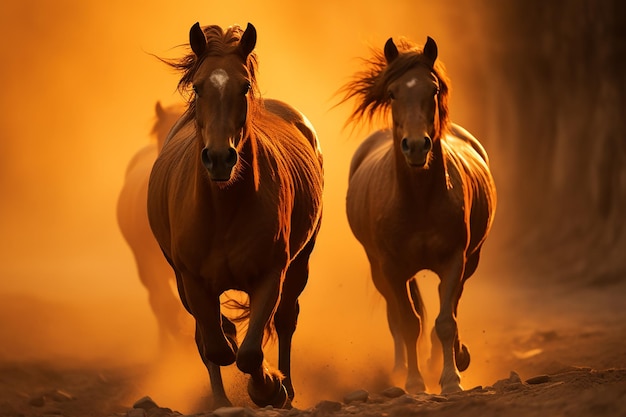The image depicts a vivid scene of three dark brown horses with white spots on their foreheads, galloping at full speed. The two horses in the foreground are prominently visible, running side by side, while a third horse is partially obscured, visible only in silhouette behind the others. The background is a rich, goldish-orange hue, blurred by the dust being kicked up by the horses as they run through a rocky, dirt-covered ground. The focus is sharply on the powerful, thick-bodied horses, emphasizing their movement and energy against the indistinct, dusty backdrop.